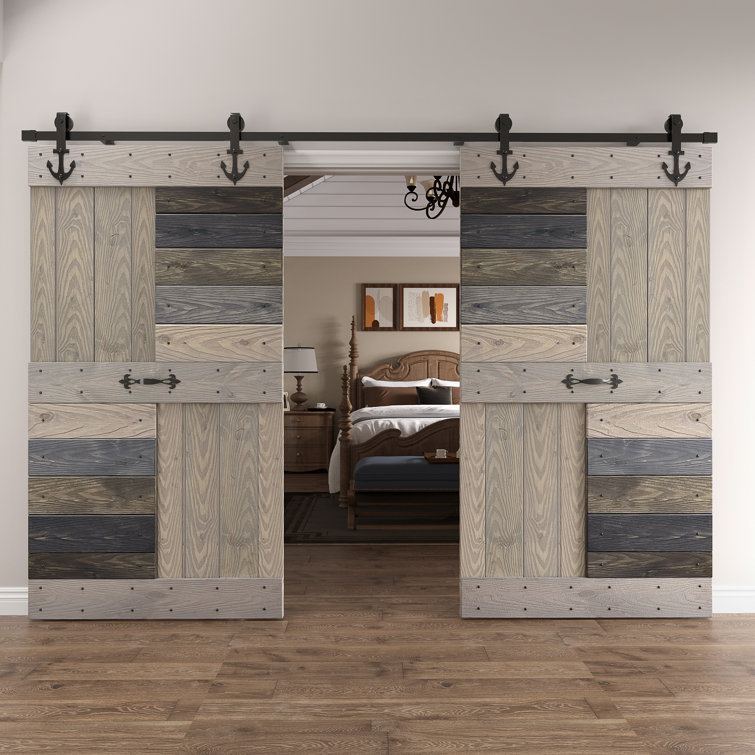This image showcases a modern bedroom with a distinct nautical and barn-inspired design. The focal point of the room is a pair of sliding barn doors with a prominent black track and hardware shaped like anchors. Each wooden door features a central brushed aluminum handle and four panels, transitioning in color from beech wood to shades of gray and dark blue. The doors open to reveal a room with medium-colored horizontal wooden plank floors and a brown four-poster bed adorned with a white bedspread, brown and white pillows, and a rounded headboard with pointed posts. At the foot of the bed is a blue-covered bench, placed on top of a gray and black carpet. The room's decor includes a wooden nightstand with a lamp boasting a white lampshade, a black chandelier hanging overhead, and tan walls adorned with white shiplap. The overall ambiance merges rustic and nautical elements into a cohesive and inviting space.